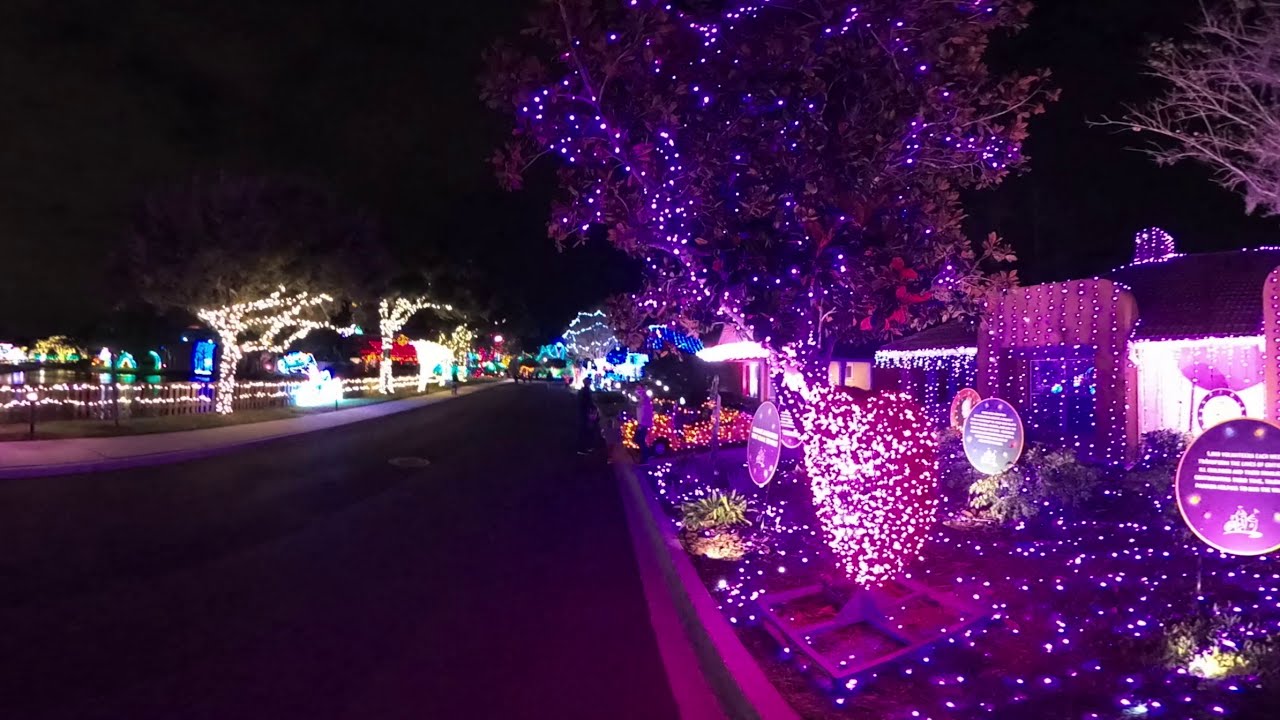The image depicts a serene, dark night landscape illuminated by an extensive display of festive lights along a straight, deserted road. On the right side of the image, several homes are heavily adorned with Christmas lights, covering bushes, trees, and the homes themselves. One prominently decorated home features a heart-shaped arrangement and displays with purple and pink lights, exuding a Valentine's Day ambiance. On the left, there's a fence beside a sidewalk and trees, all radiantly wrapped in multi-colored lights, including white, green, and blue. A miniature car also draped in purple-red lights adds a whimsical touch. A solitary person is visible, one house down from the camera, seemingly admiring the vibrant light display.